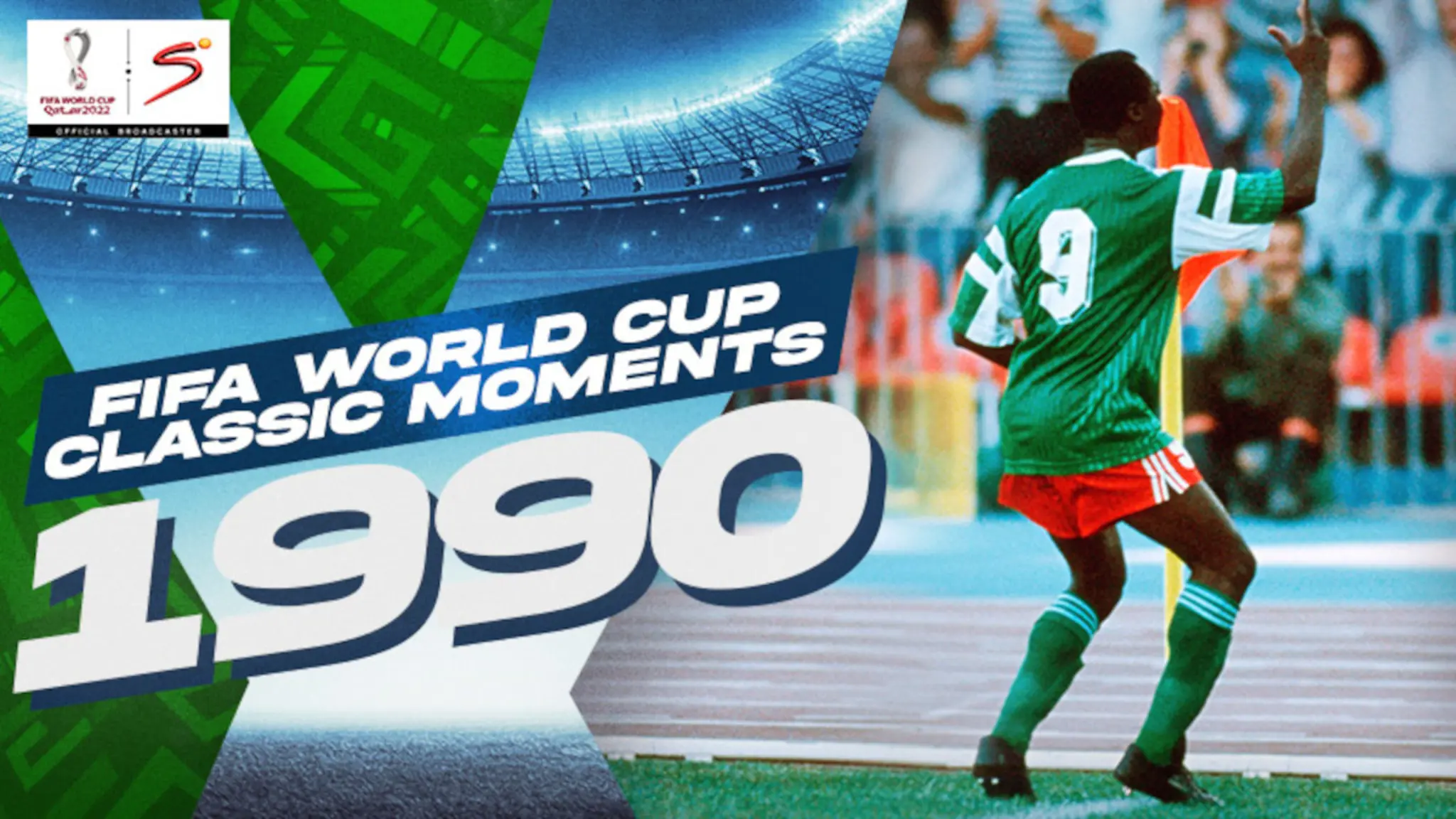This ad banner for FIFA World Cup Classic Moments 1990 features large, white, italicized lettering on the left side, stating "FIFA World Cup Classic Moments" against a stylized blue and green stadium background. At the top left corner, a smaller blue box includes the FIFA World Cup logo with an 'S' shaped emblem and the words "Official Broadcaster" in black. On the right side of the image stands an action-shot of an African-American soccer player with his back to the viewer. He is wearing a green jersey adorned with the number nine in white, blue shorts, knee-length green socks with white stripes, and black cleats. His right arm is raised in the air, and a blurry audience is visible in the distance, giving the scene a dynamic and exciting atmosphere. The prominent colors in the image are green, blue, white, red, black, and gray, enhancing the vivid and vibrant depiction of this classic football moment.